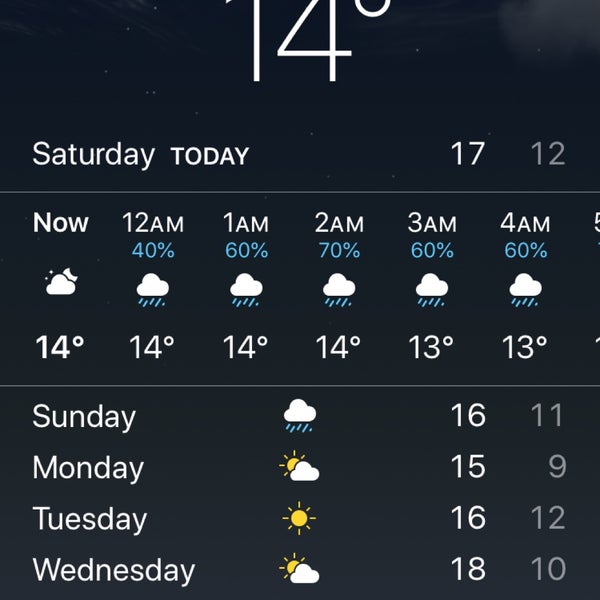A partial screenshot of an iOS weather app interface is shown, but the complete app or location name is not visible. The screenshot displays the current temperature as 14 degrees, and it's ambiguous whether this is in Fahrenheit or Celsius. Visible on the screen are columns signifying different times and their corresponding weather conditions for a Saturday. The times listed start from 'now' through several hours of the following morning, including 12 a.m., 1 a.m., 2 a.m., 3 a.m., and 4 a.m. Each time column shows precipitation percentages and accompanying weather icons indicating rain (with values such as 40%, 60%, and 70%) and temperatures around 14 or 13 degrees.

Additionally, the forecast for the next four days is shown. For Sunday, there is a rain cloud icon with a temperature of 16 degrees. Monday shows a partly cloudy icon and a temperature of 15 degrees. For Tuesday, the icon displays a sun with a temperature of 16 degrees. Similarly, Wednesday has a partly cloudy icon with a temperature of 18 degrees.